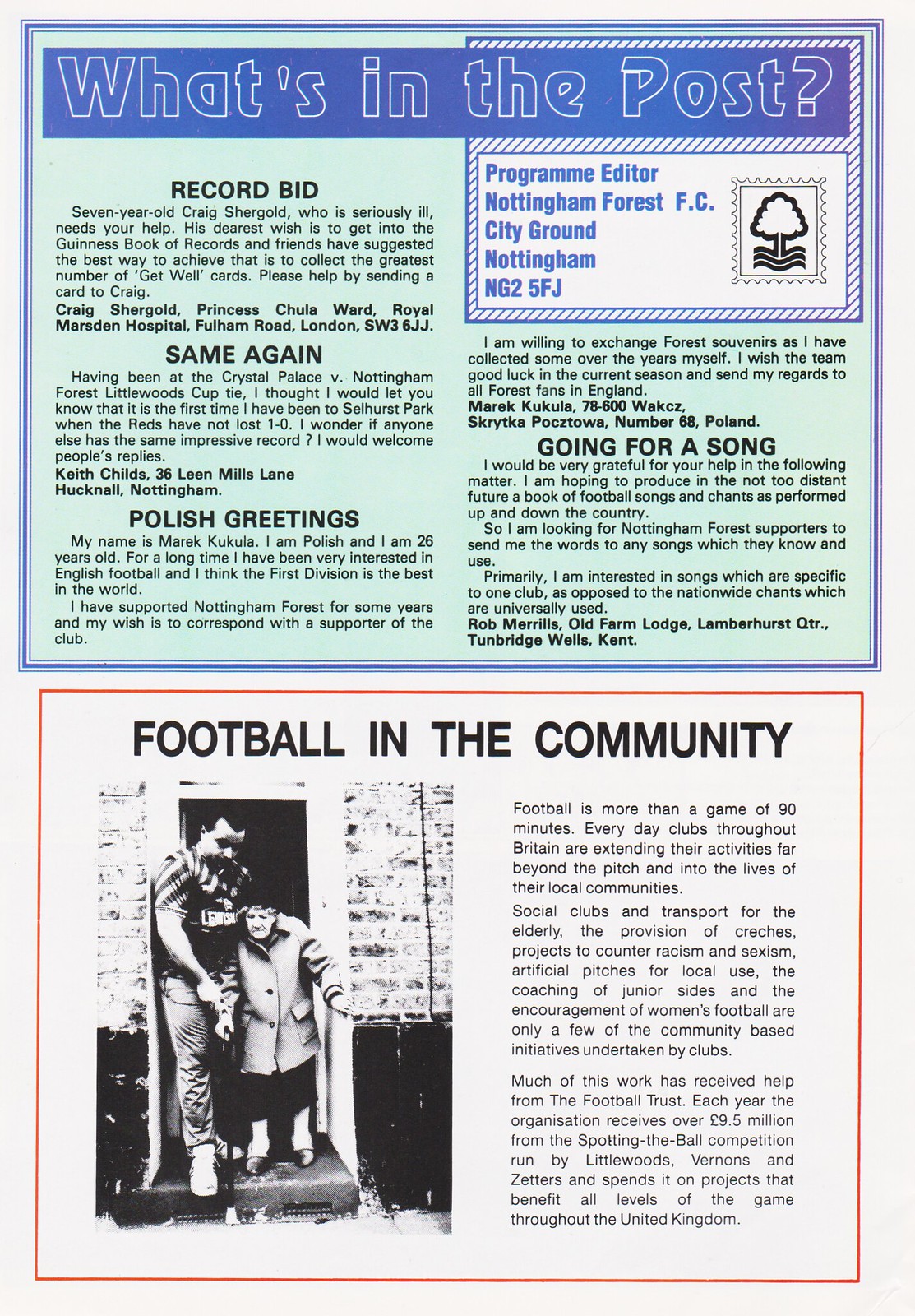The image is a large, tall poster divided into two distinct halves. The top half features a very light blue background bordered in dark blue, with a dark blue header stating "What's in the Post?". Below the header, in prominent black lettering, it reads: "Record Bid: Seven-year-old Craig Shergold, who is seriously ill, needs your help. His dearest wish is to get into the Guinness Book of World Records. Friends have suggested the best way to achieve this is by collecting the greatest number of get well cards. Please help by sending a card to Craig Shergold, Princess Chula Ward, Royal Marsden Hospital, Fulham Road, London, SW3 6JJ."

The bottom half of the poster transitions into a different topic with the title "Football in the Community." This section includes a picture of an elderly woman with a man wearing a soccer jersey. The text explains how football clubs throughout Britain are extending their influence beyond the pitch and into local communities, setting up social clubs and transport for the elderly, providing creches, tackling racism and sexism, creating artificial pitches for local use, coaching junior sides, and encouraging women's football. These community-based initiatives are supported by the Football Trust, which receives over £9.5 million annually from the Spotting the Ball competition, funded by Littlewoods, Vernons, and Zetters, and allocates these funds to various projects benefiting the game at all levels across the United Kingdom.